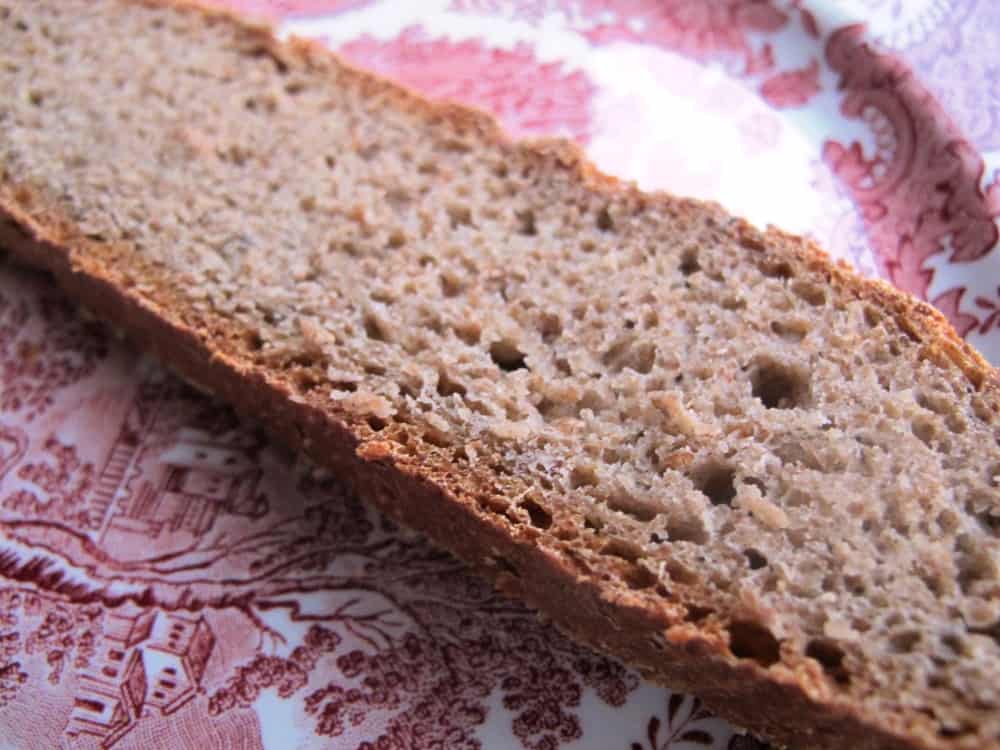In the foreground of the image is a close-up of a cut slice of homemade bread, likely sourdough or wheat, as suggested by its characteristic holes and light brown center with a darker brown crust. The slice stretches diagonally from the top left corner to the bottom right, dominating the composition. The bread is placed on a round plate that features a red and white color scheme. The plate is adorned with intricate illustrations, including trees and houses, resembling a Victorian-era or traditional Chinese porcelain design often seen in the blue and white willow patterns. The detailed drawings are especially clear on the lower left side of the image, where you can discern a large tree with a house underneath it and other architectural elements around it. The table beneath the plate is covered in a red and white cloth, adding to the rich, textured background of the scene.